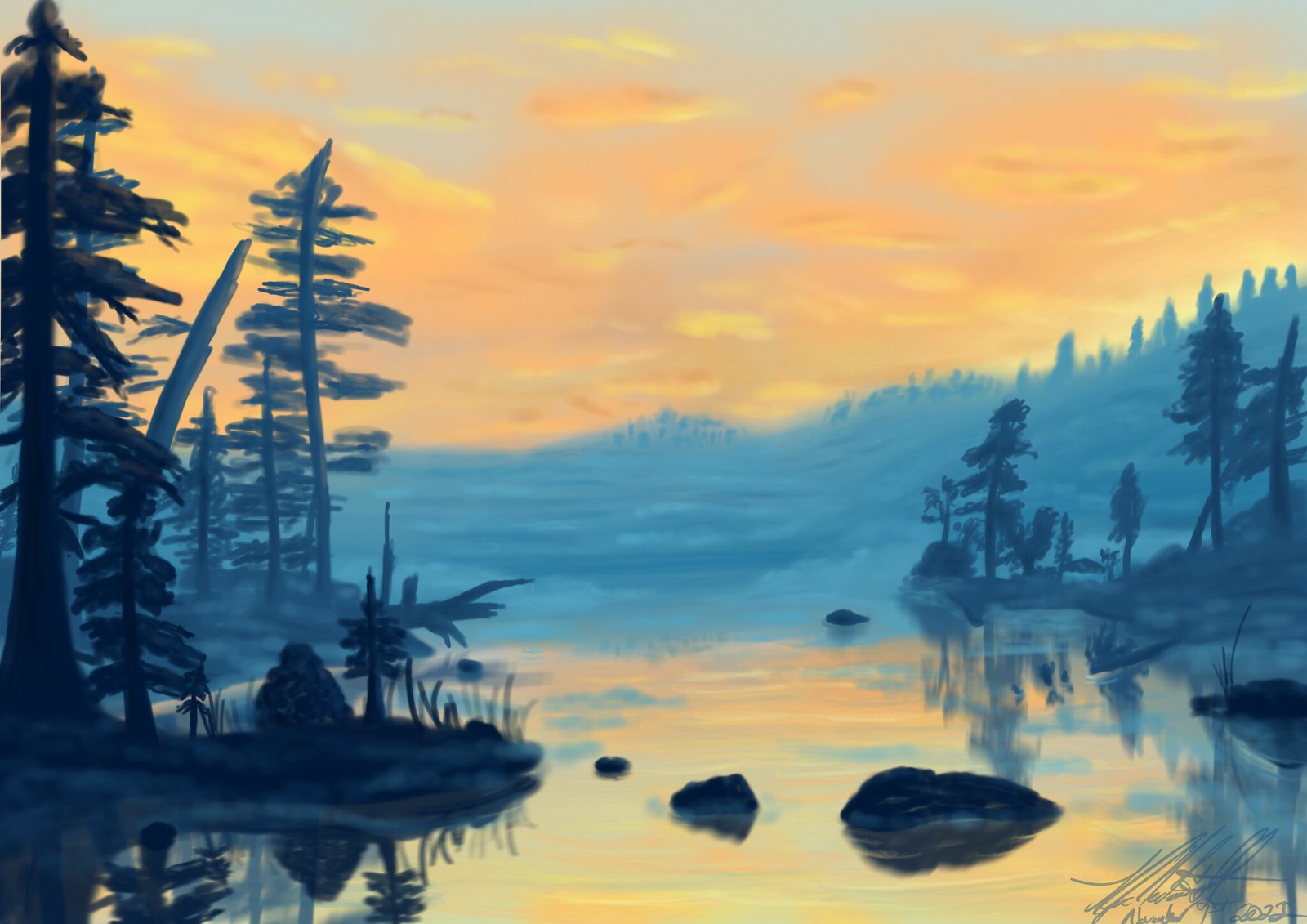This captivating oil painting depicts a serene mountain lake during the early hours of sunrise. The majestic mountains rise prominently in the background, their peaks gently kissed by the first light of day. The sky above is an enchanting blend of soft orange hues, with the underside of the clouds brilliantly illuminated by the morning light. A trace of blue sky is visible at the very top of the painting, adding a touch of coolness to the warm tones.

The tranquil water of the lake mirrors the vibrant oranges and subtle blues of the sky, creating a mesmerizing reflection. Scattered across the water are a few rocks, adding texture and depth to the scene. To the left, a cluster of towering trees, primarily conifers, stands tall alongside a few fallen snags, signifying both life and decay. This area is connected to the main scene by a small spit of land, where additional trees and shrubs cast their reflections on the water's surface.

On the right side of the painting, another spit of land extends into the distance, also adorned with trees whose reflections dance on the water. Near this area, there is an indistinct object that could possibly be an animal or a small structure, shrouded in mystery.

In the bottom right corner, the artist has signed and dated the painting in cursive. While the exact name is unclear, it appears to contain a couple of L's and a T, with a possible initial M. The painting is dated 2022, indicating its recent creation.